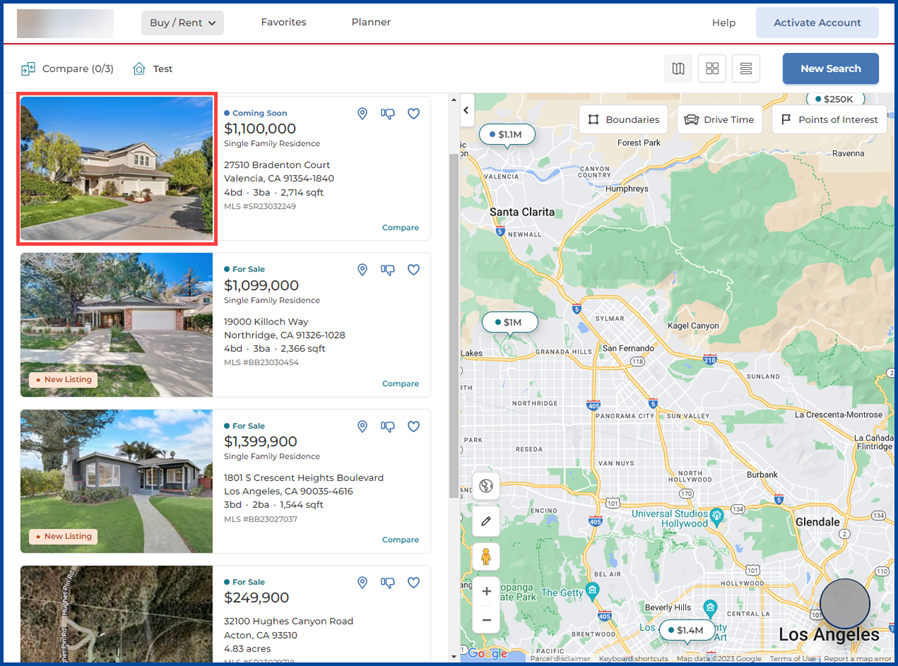A detailed and cleaned-up caption for this image could be:

"This screenshot from a real estate website features a user interface with a white background outlined by dark navy blue lines. At the top of the page, there is a white header. The upper left corner includes an obscured section within a rectangle, and next to it is a gray rectangular button with the text 'Buy / Rent' in black font, accompanied by a downward arrow indicating a drop-down menu. To the right of this button are the menu options 'Favorites,' 'Planner,' and 'Help,' each in black font. Additionally, there is a blue button on the far right with darker blue text that reads 'Activate Account.' 

Below this header, a red line separates the top menu from the property listings section. There are four property listings in total. The first listing is prominently displayed with the header 'Coming Soon.' The details for this property include a price of $1,100,000 for a single-family residence located at 7510 Brandington Court, Valencia, California, 91354-1840. The property description states it has four bedrooms, three bathrooms, spans 3,714 square feet, and the MLS number is SR23032249. Users can choose to downvote, heart, or compare the listing using icons provided next to it."